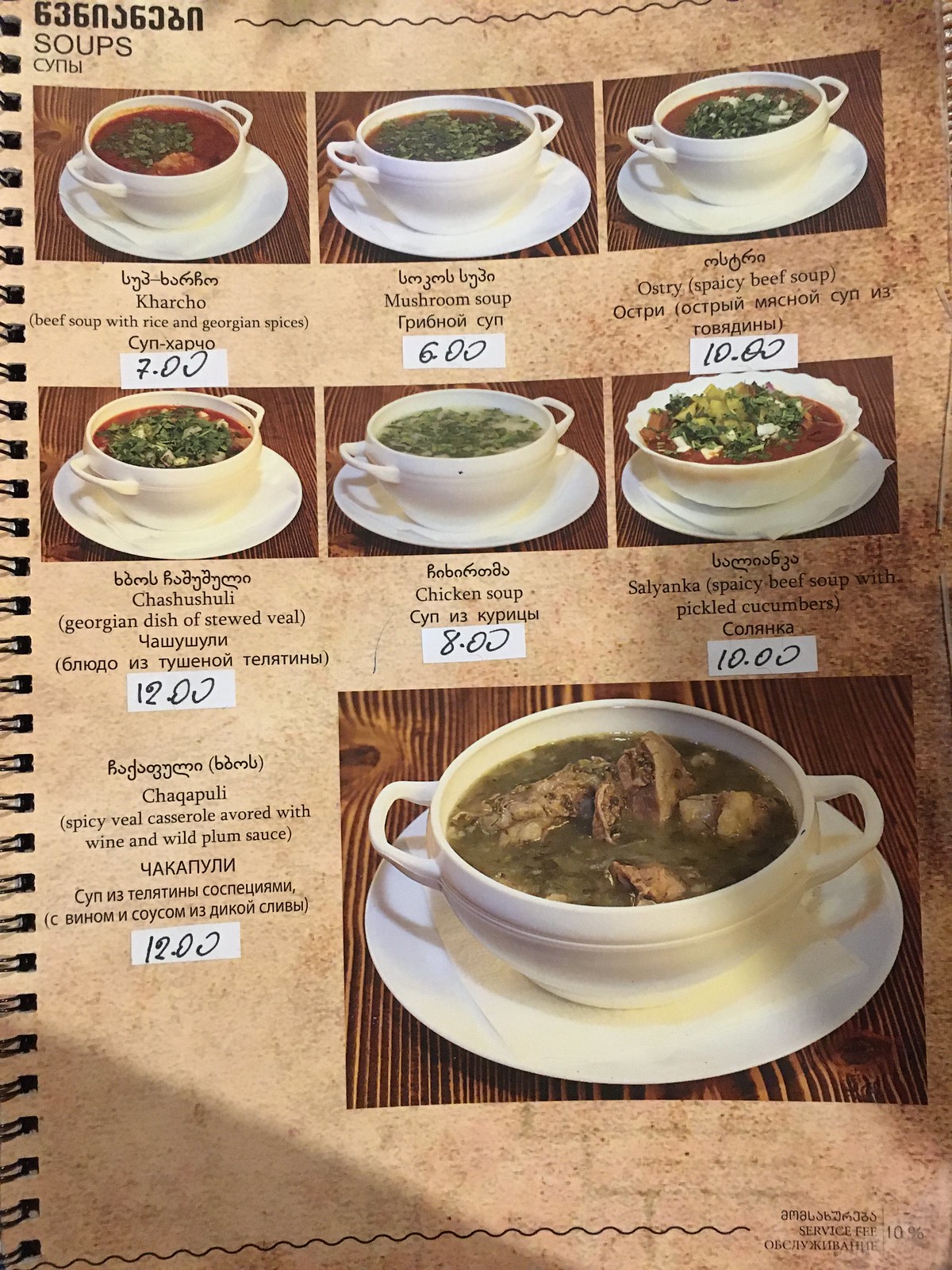The image showcases a clearly arranged menu featuring various soups served in distinctive white bowls, each adorned with dual handles on either side. The menu's top section displays six individual soup items in smaller images, while a more prominent image of a casserole appears at the bottom.

At the top of the menu, the header reads "Soups," suggesting a variety of flavorful options. Each item is accompanied by its name, a brief description, and its respective price. The descriptions are partly in a different language, likely Georgian, enhancing the menu's exotic appeal. 

1. **Karcho** - Priced at $7, this is a beef soup with rice and Georgian spices. It appears red in color with a garnish of green chives.
2. **Mushroom Soup** - This soup costs $6 and is characterized by its brownish hue, adorned with green chives.
3. **Austri** - A spicy beef soup priced at $10, also brownish in color with white pieces and a sprinkle of green herbs.
4. **Chashuli** - Described as a Georgian dish of stewed veal, this soup has a reddish appearance mixed with green and white pieces.
5. **Chicken Soup** - Available for $8, this classic soup is whitish with green flakes scattered throughout.
6. **Selyanka** - A spicy beef soup with pickled cucumbers, costing $10. It is red with green and white pieces.

The larger image at the bottom features:

7. **Tchakapuli** - A spicy veal casserole infused with wine and wild plum sauce, costing $12. This dish is green in color with visible chunks of meat.

Overall, the menu presents a diverse range of Georgian-inspired soups and a casserole, each distinctively garnished and priced, promising an array of rich flavors and culinary delight.